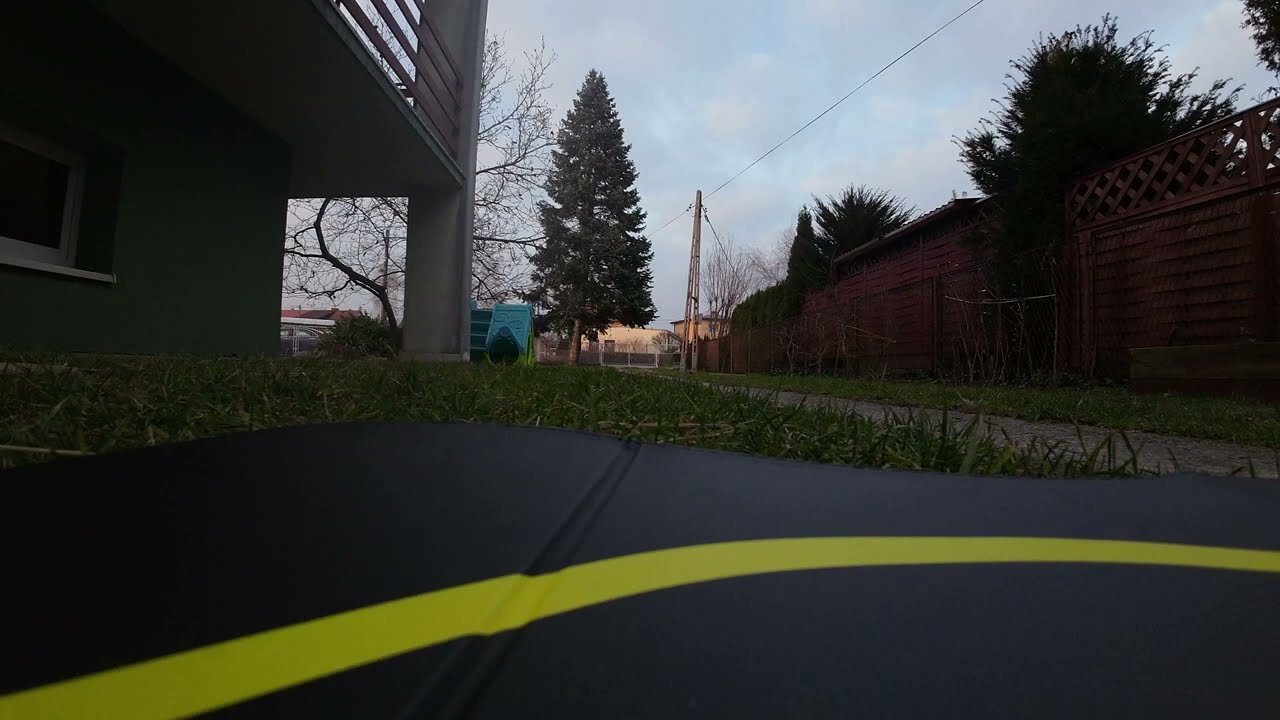The image captures a tranquil scene during the twilight hours, just after sunset, with a fading blue sky casting a dim light over the surroundings. Central to the picture is a large, dark green pine tree dominating the background, with buildings flanking it on all sides. On the left, the closest building features a stone facade and a partly visible second-story balcony, while a white-framed window can be seen on its dark green exterior. Directly in front of this building lies a grassy patch, followed by a circular asphalt area marked with a prominent yellow stripe extending from the bottom left corner and curving across the midground. The asphalt and grass are bordered by a darker, tarmac area.

To the right of the pine tree, a brown fence stretches, interspersed with various trees, including a leafless one indicating late winter or early spring. There is a slender pole with a power line near the tree, adding to the rustic ambiance. Additional structures, somewhat shrouded in the dim light, are visible behind the pine tree and to the sides, contributing to a serene yet slightly mysterious evening landscape. The minimal illumination enhances the interplay between natural and man-made elements, making for a compelling and detailed tableau.